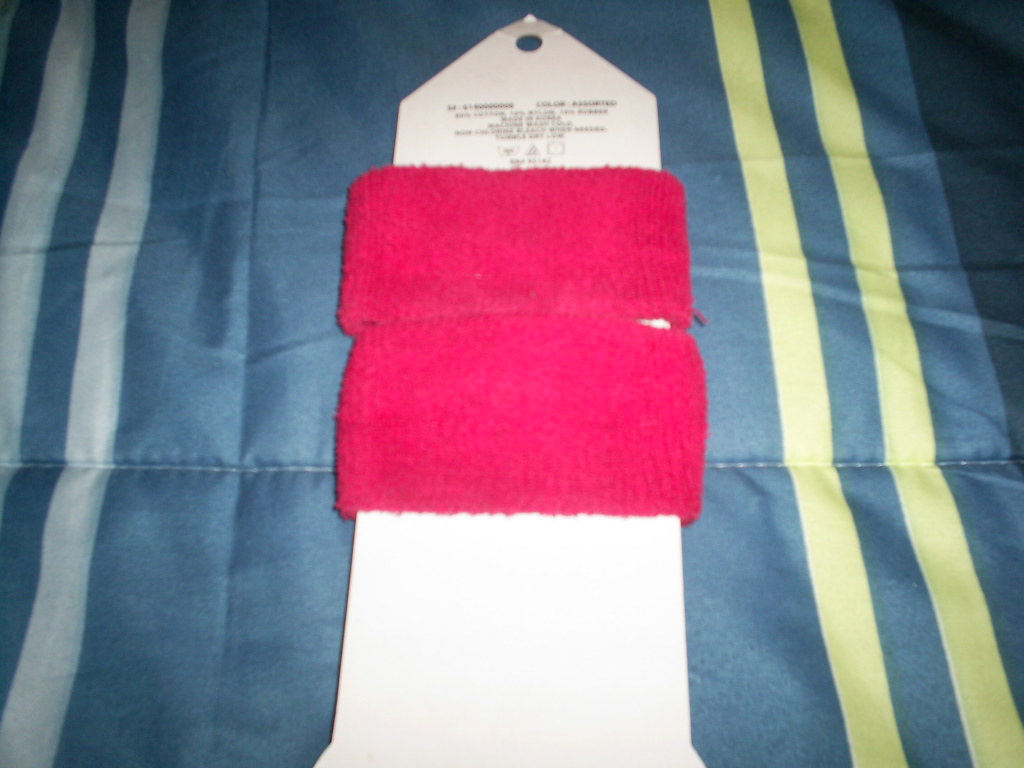The image features two dark pink terrycloth wristbands secured around a white cardboard backing, indicative of retail packaging. The cardboard has a triangular top with a hole for hanging and black text at the top. These wristbands are positioned on a blue quilted fabric backdrop that resembles a bed comforter or silky pillowcase. The background fabric includes two long white vertical stripes on the left and two long yellow vertical stripes on the right, adding a layered texture to the scene.